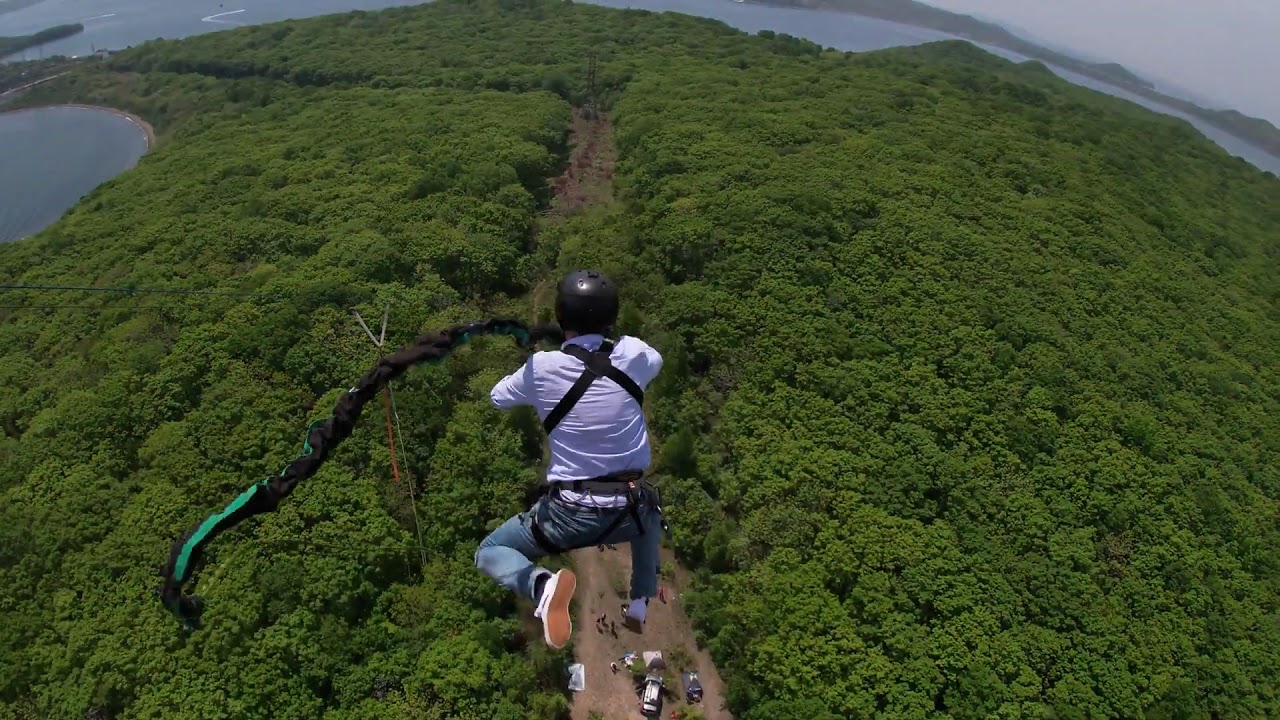The image captures a dramatic moment of a man, clad in blue jeans, a white long sleeve shirt, a black helmet, and a black harness, diving through the air from a significant height. A black parachute with green accents is deployed in front of him, suggesting he's paragliding. He is suspended high above a lush, heavily forested landscape, with various vehicles parked in a clearing directly below, perhaps waiting for him to land. The expansive scene stretches to a distant horizon featuring lakes, hills, and mountains. The sky is particularly striking, with murky dark gray clouds encroaching from the top right corner, adding a sense of impending weather changes. The overall impression is one of adventurous thrill amidst the vast and scenic natural beauty.